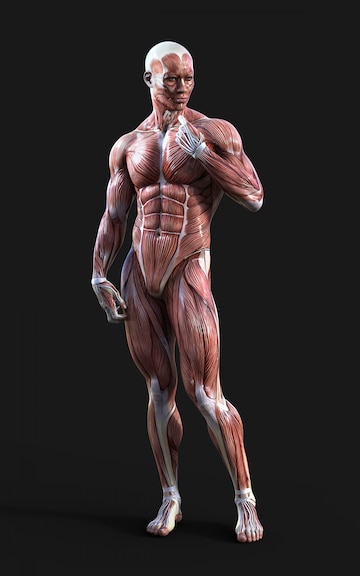This is a detailed medical representation of a highly muscular male figure, standing against a stark black background. The figure is devoid of skin, showcasing an intricate display of the body's muscular and skeletal anatomy. The muscles are vivid and well-defined, with a reddish hue, highlighting the abs, pecs, and other major muscle groups. The figure's eyes are visible, and the front of the skull is exposed, transitioning from white at the top to red facial muscles below. Additionally, the shin bones, kneecaps, tops of the feet, and the back hand bones are prominently white, contrasting sharply with the muscle tissue. The figure is oriented to the right, not looking directly at the camera, and appears in three-dimensional form, possibly as part of a medical diagram or educational tool. The overall effect is not frightening but rather an informative and beautiful portrayal of human anatomical structure.